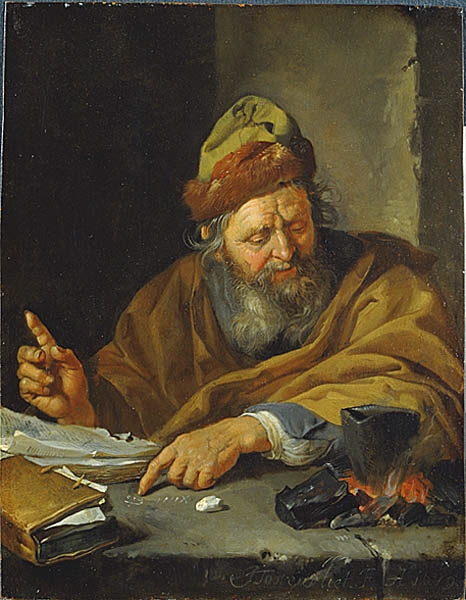The image is a colorful painting with predominantly muted tones of dark brown, black, gray, and dark green, contrasted by lighter shades of golden brown. It depicts an old man, seemingly deep in thought, sitting next to a rough, concrete-like table. He is surrounded by various objects: a stack of white papers with writing on them, a closed book, and a piece of white chalk used to draw on the stone near his hand. A small fire burns on the table, with a dark chalice or cup heating in the flames. The man wears a golden-brown robe and a green and brown hat, and appears to be contemplating or counting something.